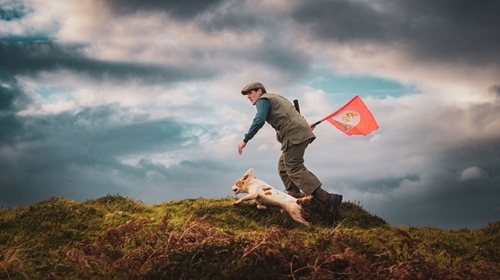In this small rectangular horizontal image, a boy is running along the top of a rugged, grassy hill with his loyal dog at his side. The boy, who is dressed in earthy brown hiking boots and clothes, carries a red flag with a white circle, which hangs out of his backpack. His hand is bare, and he is not wearing a hat, contrasting with the dog's striking appearance. The dog is predominantly white with brown spots and tan markings on its head and tail. The scene has an intense backdrop of dark, ominous clouds interspersed with patches of blue and white, giving the sky a dramatic, almost foreboding atmosphere.